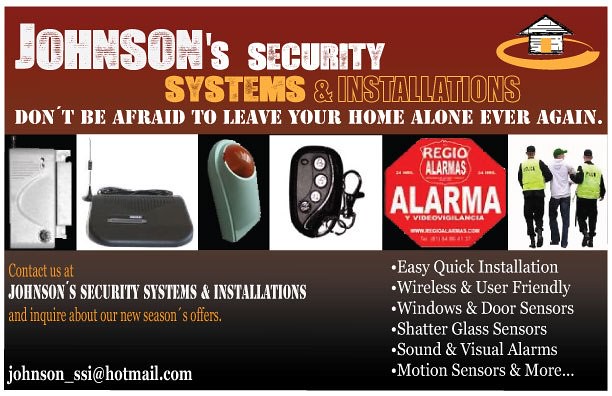This advertisement for Johnson Security Systems and Installations is split into three distinct sections with a rich and varied color scheme. The top of the image features a deep red background, with text in contrasting colors. "Johnson Security" is prominently displayed in white, followed by "Systems and Installations" in a striking yellow-gold-orange hue. Below this, in white capital block letters, the tagline reassures homeowners: "Don't Be Afraid to Leave Your Home Alone Ever Again." In the top right corner, a white sketch of a house with a yellow door is encircled by a yellow ring, adding visual interest to the upper section.

The middle section showcases a series of six images, displaying various security tools and devices. These include a silver object on a black background, possibly a piece of security hardware; a device resembling a Wi-Fi router on a white background; a white object with a prominent red light; a key fob; a red hexagon sign reading "ALARMA" in white; and finally, an image of two police officers in greenish jackets and black pants, carrying a man in a white sweatshirt and blue jeans.

The bottom section transitions to a gray-to-black fade, providing contrast to the top and middle sections. Here, it invites potential customers to "Contact us at Johnson Security Systems and Installations and inquire about our new season's offers," with the email address johnson_ssi@hotmail.com displayed in the bottom left. The right side of this section lists the benefits and features of their services in white bullet points: "Easy, quick installation, wireless and user-friendly, windows and door sensors, shatter glass sensors, sound and visual alarms, motion sensors, and more."